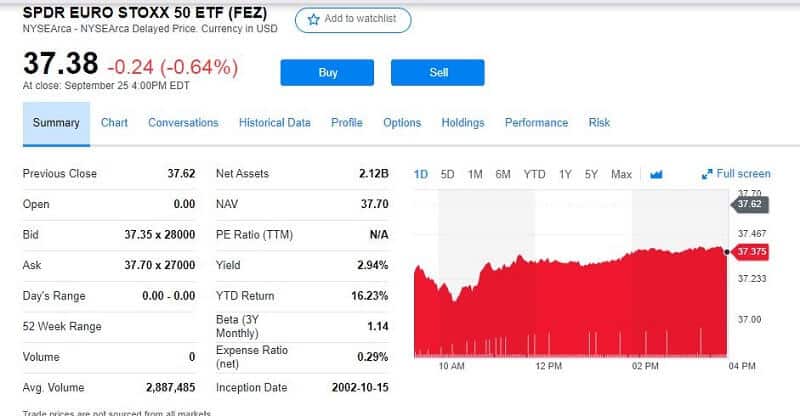This image is a screenshot of a financial stock trading platform displaying detailed information about the SPDR EURO STOXX 50 ETF. The page highlights that the current stock price is $37.38, showing a decrease of $0.24, equivalent to a 0.64% drop in its total value. The interface provides buy and sell options, indicating that the user is currently browsing the stock details. 

The screenshot reveals various data points, including the stock's average trading volume, bid price, ask price, opening price, and the previous closing amount. Additionally, a predominantly red line graph is shown, illustrating the stock's declining performance. The background of the page is white, and in the top left-hand corner, the stock is clearly identified as SPDR EURO STOXX 50 ETF. 

This comprehensive display offers a thorough insight into the stock's current market situation.